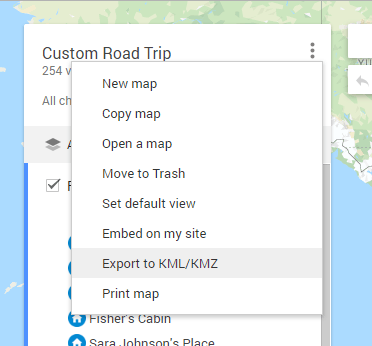The image displays several overlapping windows superimposed on a map interface. The most prominent window in the center features various options, including "New map," "Copy map," "Open a map," "Move to trash," "Set default view," "Embed on my site," "Export to KML/KMZ," and "Print map" in black text on a white background. Behind this primary window lies another window titled "Custom Road Trip," partially obscured, with the number 254 and three vertical dots in the upper right corner visible. At the lower part of the image, still partially visible, are labeled locations such as "Fisher's Cabin" and "Sarah Johnson's place." The map, which forms the backdrop, reveals hints of blue water and green landforms, though the specific geographic details remain concealed due to the overlaying windows. The overall color scheme is dominated by white, complemented by black text and elements of blue and green from the underlying map.